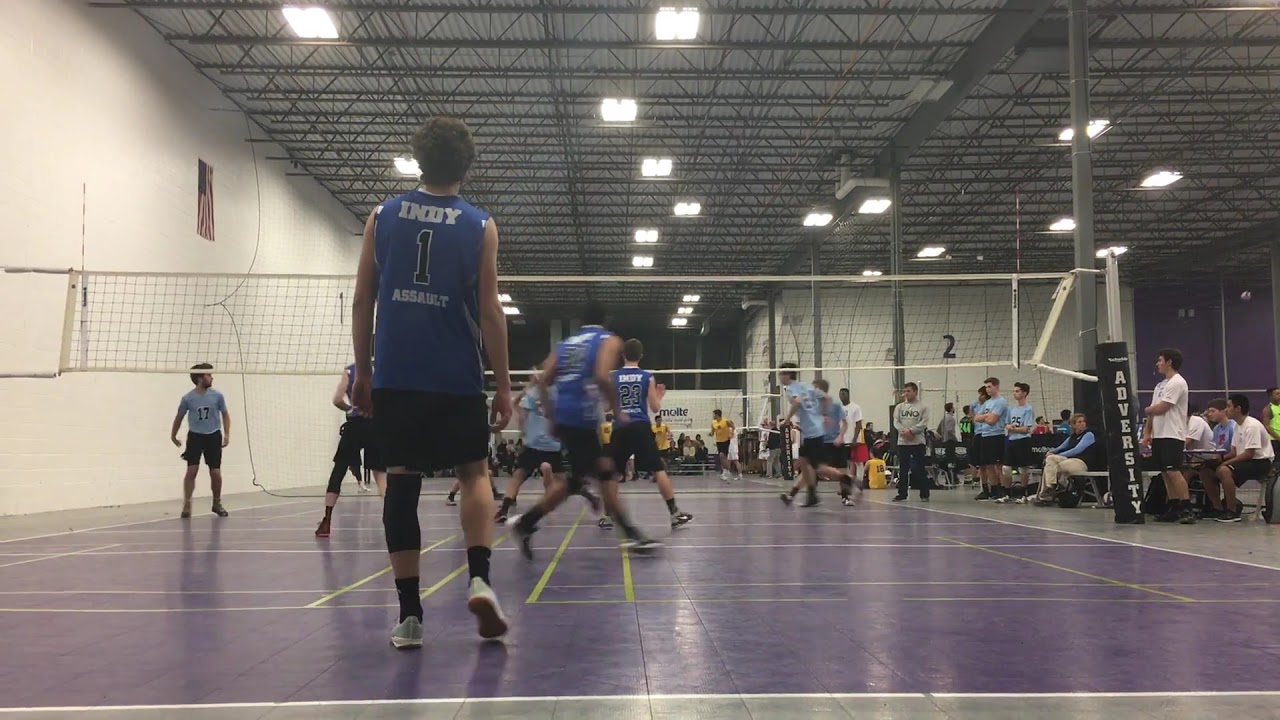This photograph captures an indoor high school men's volleyball game. The scene is viewed from one end of the court, slightly below head level, emphasizing the action and the structures above. The court itself has a purpley gray surface marked with official lines. The team closest to us is wearing dark blue jerseys with black shorts; prominently featured is a player just left of center with dark hair, donning a jersey that reads "Indy 1 Assault." Other members of this team also sport similar jerseys. Their opponents are dressed in light blue shirts and black shorts.

The gymnasium is spacious, with high ceilings that expose metal rafters and bright lights illuminating the court below. The left side of the image features a white wall, while the right side is lined with spectators engrossed in the match. In the background, additional figures can be seen, some of whom might be players from another concurrent game, contributing to the lively and bustling atmosphere of the event.